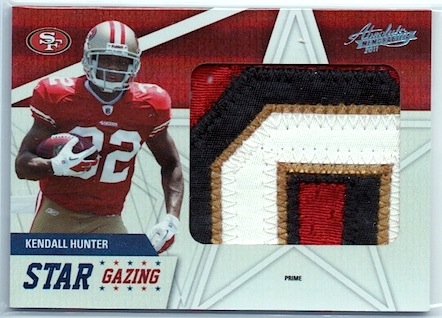This color photograph showcases a detailed piece of sports memorabilia for the San Francisco 49ers, featuring a prominent image of football player Kendall Hunter wearing his red jersey with the number 22, white gloves, and iconic gold helmet as he carries a football under his right arm. The background is decorated primarily in the 49ers' colors, red and white, with a large white star across the center. To the left of the box, there's a noticeable oval red logo with the SF emblem. Below the action shot of Hunter, his name is captioned on a blue band in white bold lettering, followed by the word "Stargazing" in a red and white pattern. An inset window towards the right center gives a peek at the embroidered stitching of the jersey inside. The top right corner of the box features a blue logo with a memorabilia slogan bearing the year 2012. Additional small black letters below the window spell out "prime," adding to the authenticity of the collectible.